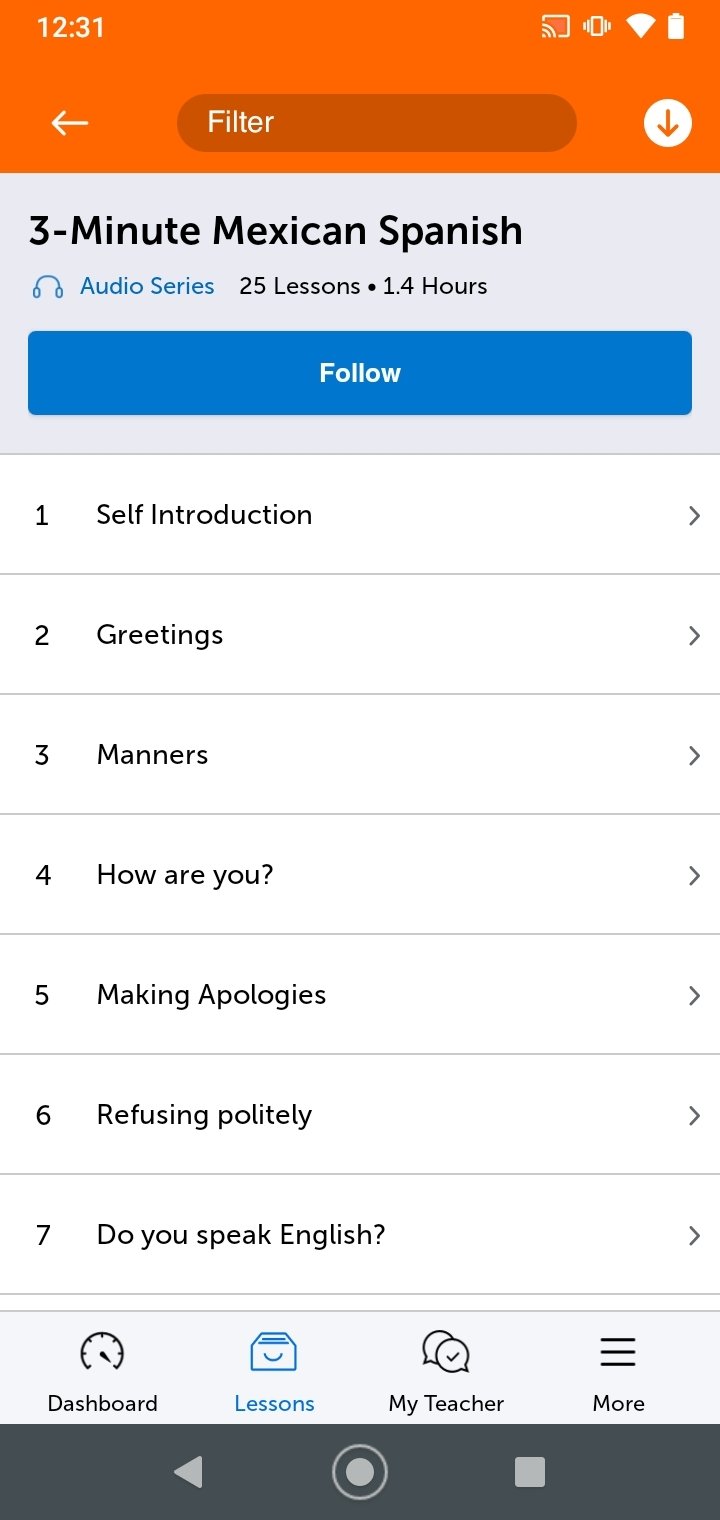**Caption:**

Screenshot of a mobile app displaying a language learning course titled "3-Minute Mexican Spanish." The course comprises 25 audio lessons, totaling 1.4 hours. A prominent blue "Follow" button appears on the screen. The course features seven sections: 

1. Self-Introduction
2. Greetings
3. Manners
4. How Are You?
5. Making Apologies
6. Refusing Politely
7. Do You Speak English?

At the bottom of the screen, a menu bar includes options for Dashboard, Lessons, My Teacher, and More, with the Lessons tab currently selected. An orange search bar sits at the top, featuring a back button, a filter icon, and a downward arrow. The phone's standard navigation buttons (back, home, and recent apps) are visible at the very bottom.